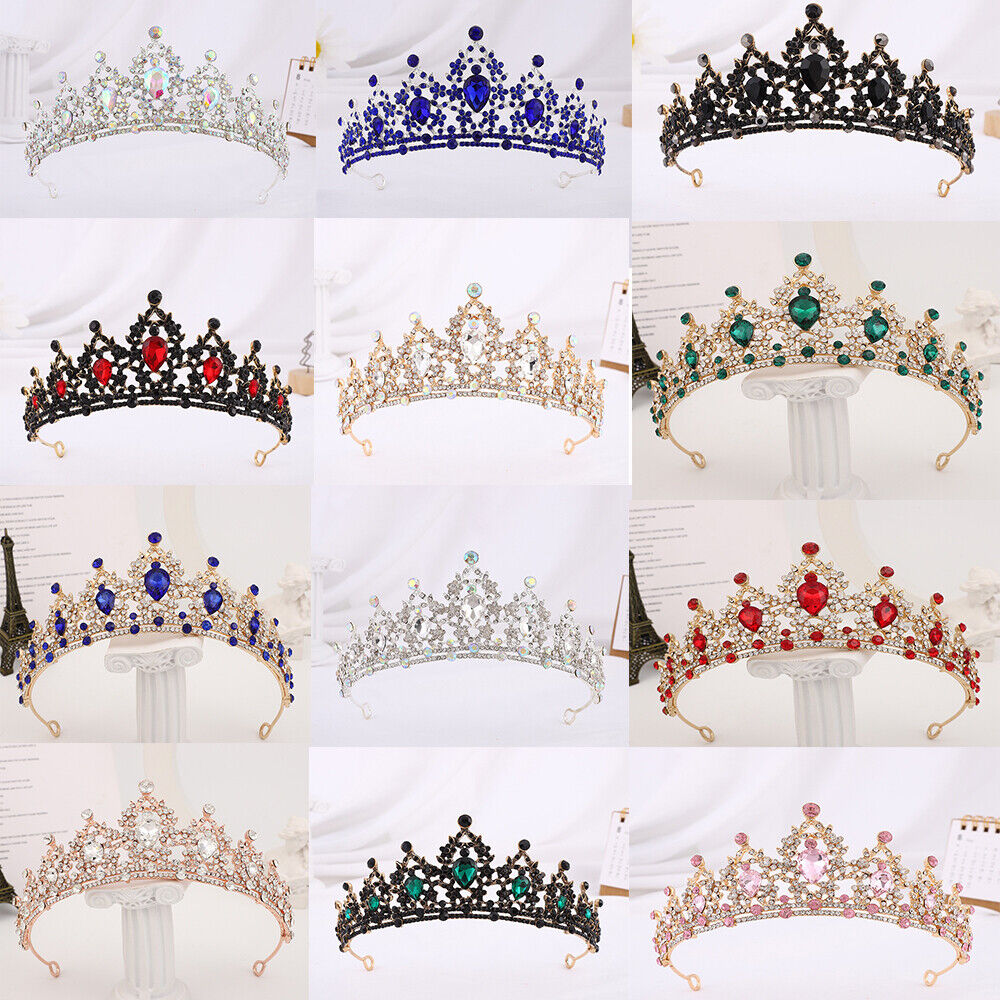The image showcases an array of 12 photographs, arranged in a grid of three rows and four columns, featuring a dazzling collection of tiaras. Each tiara is displayed against various backdrops, including curtains, pillars, and decor elements like paper with writing and a miniature Eiffel Tower. The tiaras, though similar in design, exhibit a striking variety of colors and materials. Starting from the top left, there is a tiara adorned with clear diamonds and accented by light turquoise and pink gems. Next, a tiara with vibrant blue, sapphire-like gems follows. The top right features a tiara with black and clear gems. The second row starts with a black metal tiara embellished with red gems, followed by a gold metal tiara with clear, diamond-like gems, and another gold tiara with rich emerald green gems. In the third row, we find a gold tiara with sapphire gems, a silver tiara decorated with a mix of light blue and yellow gems, another gold tiara with what appears to be clear diamonds, and a tiara featuring ruby red gems. The final row includes a tiara with pinkish gemstones set in white metal, a black metal tiara with green gems, and lastly, a gold tiara with two shades of light pink gems. Each tiara's intricate design and vibrant colors are prominent against the varied but subtly cohesive backgrounds, making for a visually captivating display.